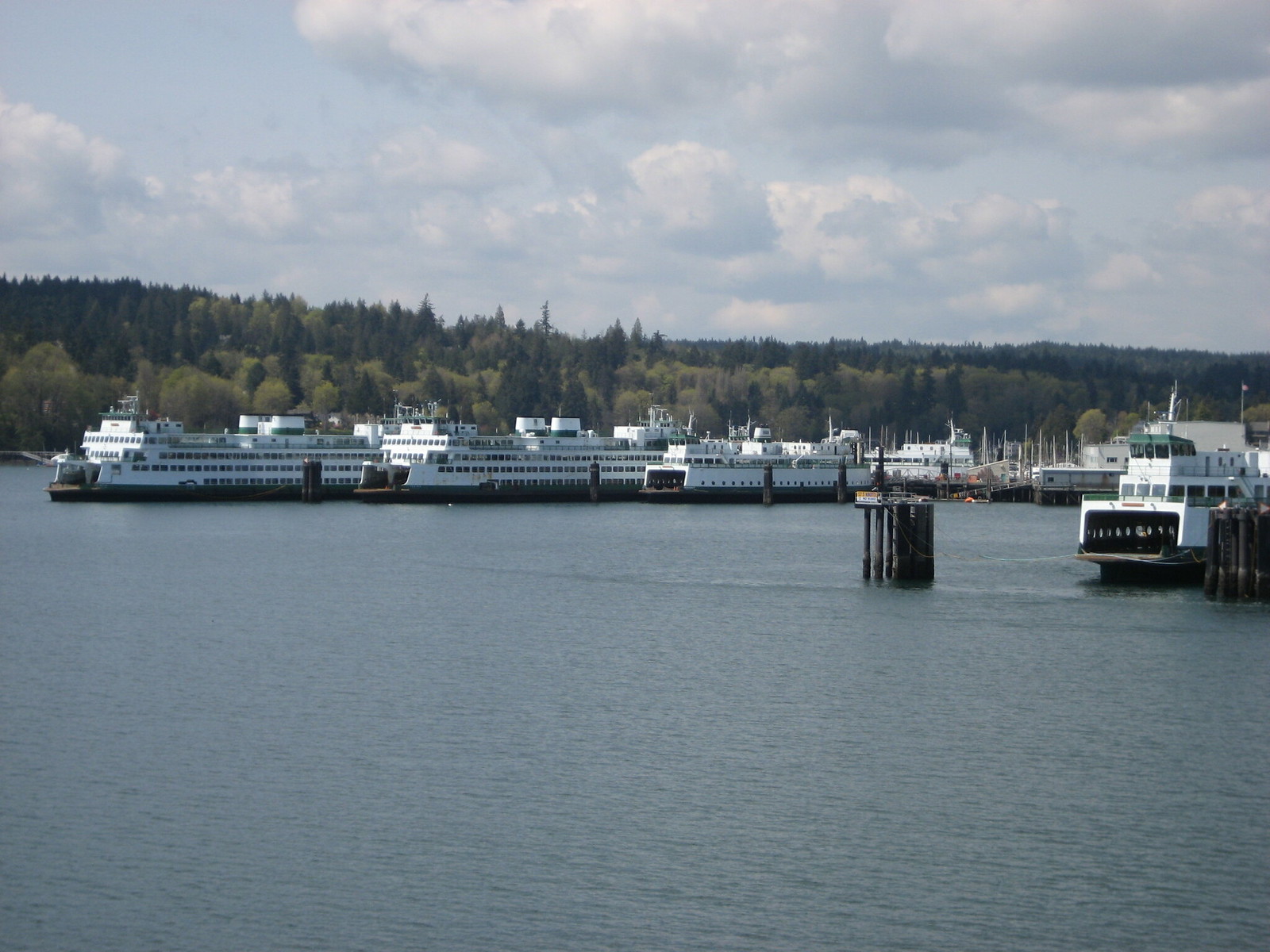The image shows a tranquil bay with several large ferry boats docked along the shoreline. These ferry boats, predominantly white with black undersides and open back ends, are lined up neatly in the water. The water itself is a deep blue, gently rippled by waves, and covers the lower portion of the photograph. In the middle, the horizon features a stretch of land densely covered with green and black trees, devoid of any buildings. Emerging from the water to the right is a small post or pole of an uncertain nature. Dominating the upper part of the image is a cloudy, grayish-blue sky with patches of light blue where the clouds have parted. The clouds are puffy and mostly gray with hints of white. The image, taken in the morning, captures the sunlight subtly illuminating parts of the boats while casting shadows on the other areas, giving a nuanced depth to the scene. The overall color palette of the photograph is subdued, with a bluish-grey exposure, lending a calm and serene atmosphere to the landscape.